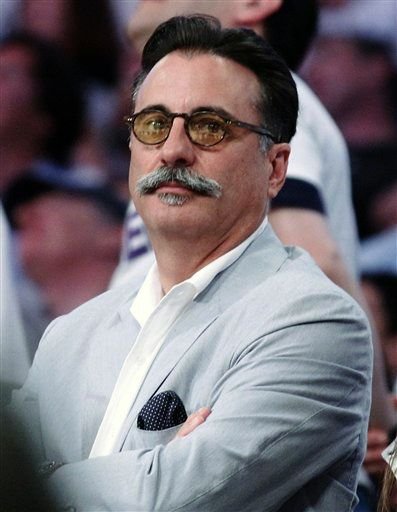The color photograph features actor Andy Garcia from his lower chest upwards, dressed in a light gray business coat over a white button-up shirt with the top buttons undone. A black handkerchief with white polka dots peeks out from his left breast pocket. Garcia's black hair is swept backward, and he sports black-rimmed circular glasses with yellow lenses. His facial hair includes a gray and black beard, mustache, and goatee. With his body oriented towards the bottom left corner of the frame, his face is directed forward with an expressionless demeanor. His arms are crossed over his chest. 

In the blurred background, multiple people appear to be looking in different directions. Directly behind Garcia stands a man in a white short-sleeve t-shirt with black trim, gazing upwards. The overall photograph has a slightly unfocused quality, particularly in the background, highlighting Garcia as the primary subject.